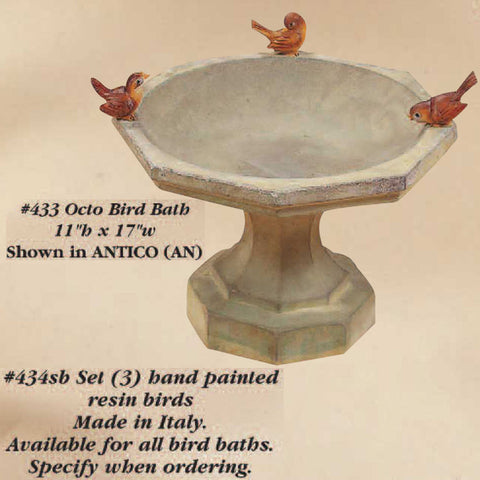The image is an advertisement for a beige octagonal bird bath set against a light brown background. The bird bath, identified as item number 433 Octo Bird Bath, measures 11 inches in height and 17 inches in width, and is shown in a finish referred to as "Antico (AN)." Atop the bird bath are three reddish-brown, hand-painted resin birds, although they appear more orange in the image and resemble sparrows. These birds, designated as item number 434SB, are made in Italy and are available as a separate set that can be added to any bird bath upon specification when ordering. The text in the advertisement is rendered in black and is located primarily in the middle and lower sections of the image, providing detailed product information.